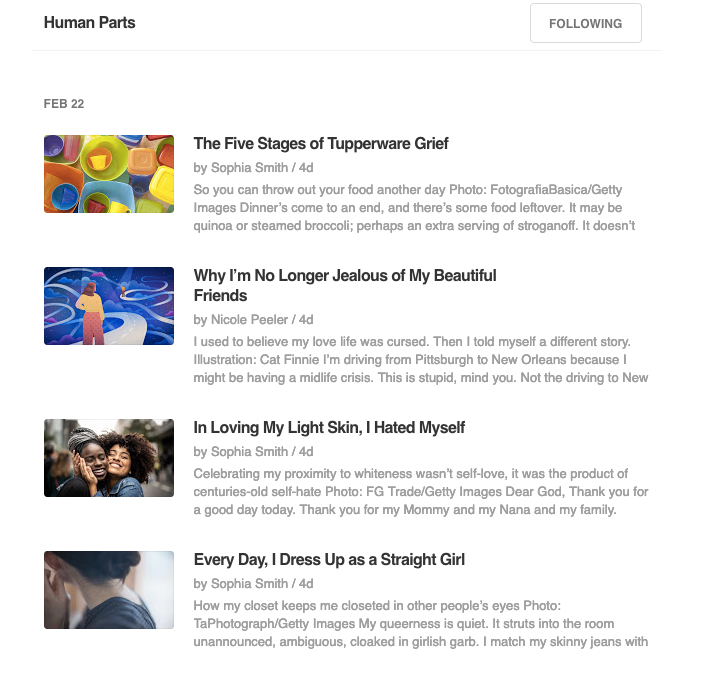The image is a detailed visual representation of a website interface. In the upper left-hand corner, the website is titled "Human Parts." On the right side, there is a box labeled "Following." The displayed date is February 22nd. 

The main feature of the webpage is an article titled "The Five Stages of Tupperware Relief," which showcases an assortment of Tupperware containers with various lids of different shapes, colors, and styles. The article appears to delve into common experiences and challenges associated with managing Tupperware. 

Below this main feature, there is a visual icon depicting a person standing at the end of what appears to be a white road or path, accompanied by squiggly lines in blue and white. The person is wearing a peach-colored top and pink pants. The accompanying text for this section reads, "Why I'm No Longer Jealous of My Beautiful Friends," followed by another statement, "In loving my light skin, I hated myself." This section is illustrated by a touching image of two Black girls, one with a light skin tone and the other with a very dark skin tone, embracing each other with their faces close together.

The final section on the webpage is titled "Every Day I Dress Up as a Straight Girl." It is illustrated by an image of a girl, focusing on her left shoulder and the back of her head. The accompanying text reads, "How My Closet Keeps Me Closeted in Other People's Eyes," providing a glimpse into the personal narrative of the author’s experiences with their sexual identity.